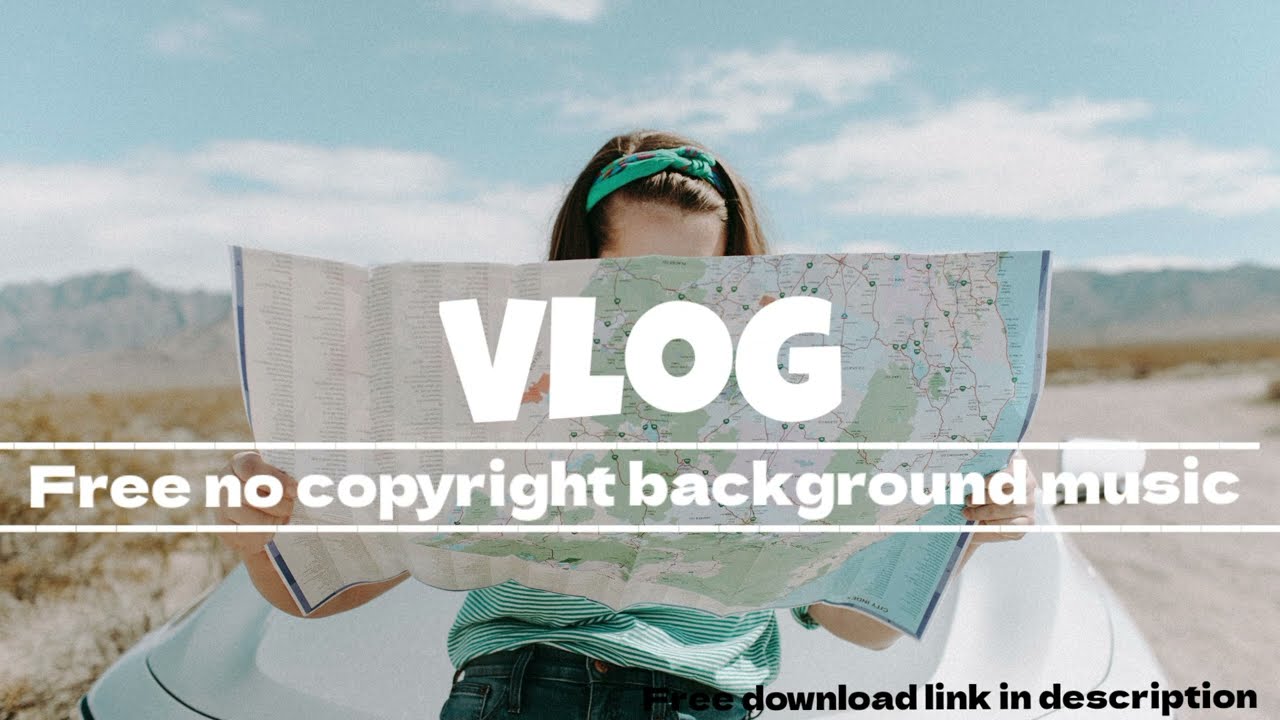In the image, a young girl with brown hair pulled back by a green headband sits on the hood of a silver car, holding a large road map that obscures her face and much of her body. She is wearing a green and white striped shirt with blue jeans. The scene is set on a desert-like dirt road with sand extending to blurred mountainous horizons and a clear blue sky. Dominating the image are large white letters spelling "VLOG," beneath which it states, "FREE, NO COPYRIGHT BACKGROUND MUSIC," framed by two white bars. At the bottom right, black text reads, "DOWNLOAD LINK IN DESCRIPTION." This image appears to be a thumbnail for a video promoting free, no-copyright background music.